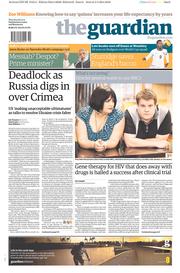**Detailed Caption for The Guardian Newspaper Image:**

The image depicts a physical copy of The Guardian newspaper. The prominent bold text "The Guardian" headlines the page. The main article features the title "Deadlock as Russia digs in over Crimea," capturing a pivotal geopolitical issue. In the top left corner, a barcode is visible, typical of printed media. Two noticeable advertisements are present:

1. One ad featuring the text "Messiah Despot Prime Minister" shows an older man, possibly Muslim, characterized by his traditional hat and a large white beard.
2. Adjacent to this figure is what appears to be an image of a soccer player, contrasting the serious tone of the article.

Within the main article, beneath the "Deadlock as Russia digs in over Crimea" headline, a photograph illustrates a fuller-figured couple leaning over a railing or table. The woman is dressed in a blouse, while the man sports a short-sleeved bowling shirt. Below this article, a broader advert promoting military service can be seen, though the small text is almost illegible due to the image's compression and JPEG artifacts. The overall quality of the image is quite poor, marked by visible compression artifacts that obscure finer details.